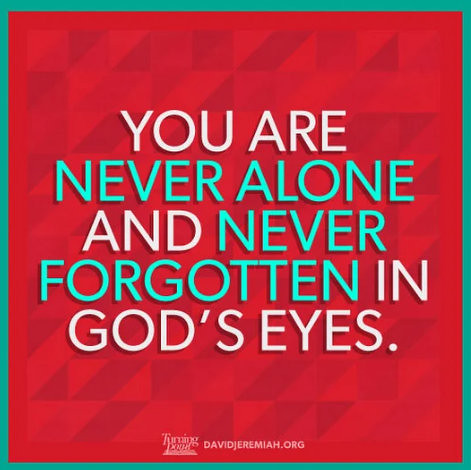This is an image of a flyer with a green border that frames all sides. The center features a red background divided into a pattern of triangles with varying shades of red, creating a textured effect. The central text reads: "YOU ARE" (in white capital letters), followed by "never alone" (in light blue). Beneath this, in white, it says "and," then continues with "never" (in light blue), followed by "forgotten" (in light blue) and "in" (in white). The final line reads "God's eyes" in white. At the bottom of the flyer, in small capital letters, the URL "DAVIDJEREMIAH.ORG" appears. To the right of the URL, there's additional text in a cursive font that's partially legible, possibly the word "Turning."